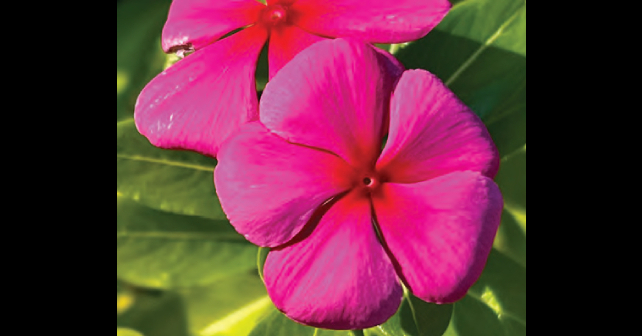The image is an extreme close-up photograph of two purplish pink flowers, each with five petals. The petals are vibrant hot pink on the outer edges, transitioning to a deep red near the center, which features a small hole. The flowers appear almost merged at the top left, suggesting a natural blending or melting effect. Behind the flowers, there are large green leaves with clearly visible veins and a main stem, slightly out of focus, creating a soft background contrast to the sharply defined flowers. The sunlight highlights parts of the leaves, casting subtle shadows and adding depth to the composition. The flowers dominate the central part of the image, with no text to identify their species, offering a striking and detailed natural scene against a stark black background.